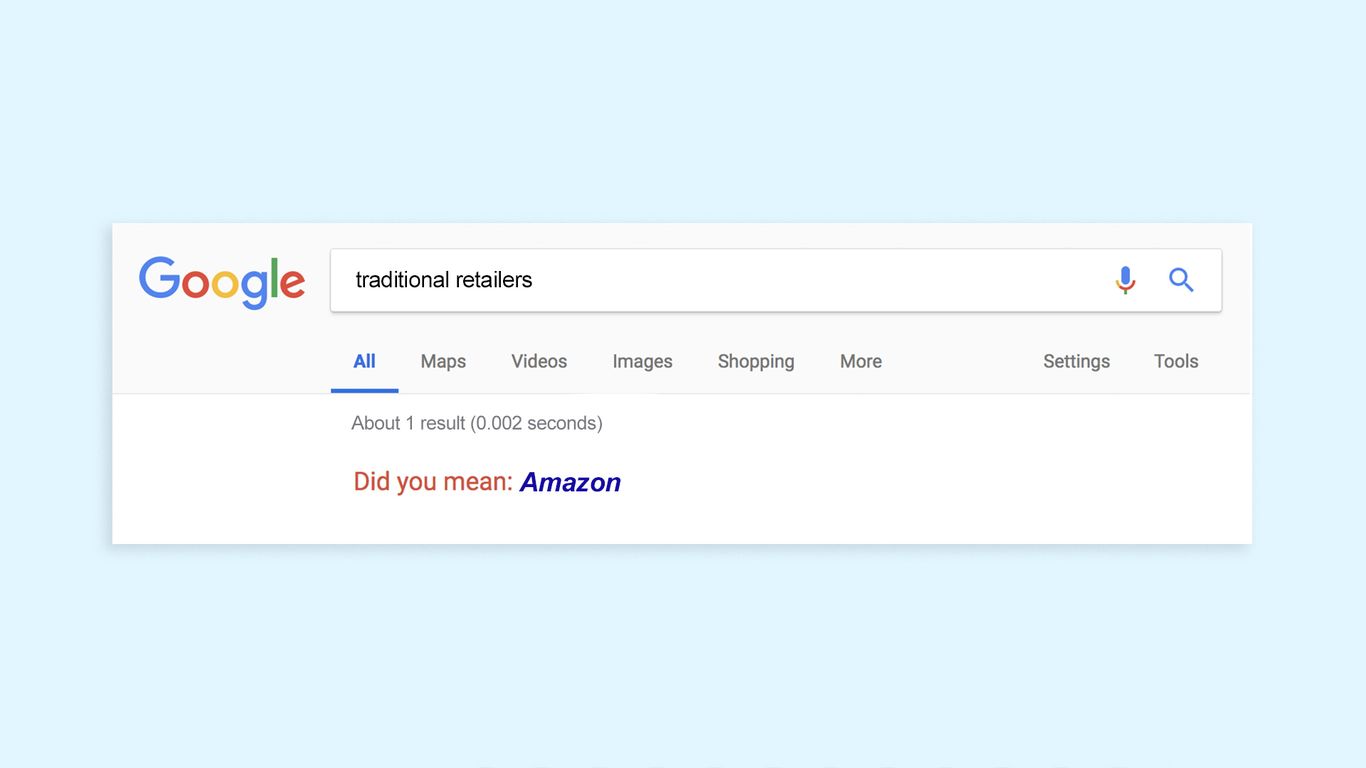The image features a light blue background reminiscent of a clear sky. In the foreground, there is a smaller rectangular box that appears to be a screenshot of a Google search interface. Positioned in the upper left corner of the box is the iconic Google logo. Below the logo, the search query "traditional retailers" is displayed within the search bar.

To the right of the search bar are two icons: a microphone icon (indicating voice search) and a magnifying glass icon (the search button). Beneath the search bar, a set of tabs includes options such as "All," "Maps," "Videos," "Images," "Shopping," and a few more, along with "Settings" and "Tools." The "All" tab is currently highlighted.

The search results indicate "about 1 result (0.002 seconds)." Directly below this, in red text, Google provides a suggestion saying, "Did you mean: Amazon." This suggests that Google might be hinting at Amazon as a popular alternative or related search for the term "traditional retailers."

The overall composition of the image effectively depicts a digital search, highlighting the interface and features of a standard Google search page, while the serene light blue background provides a visually appealing contrast.